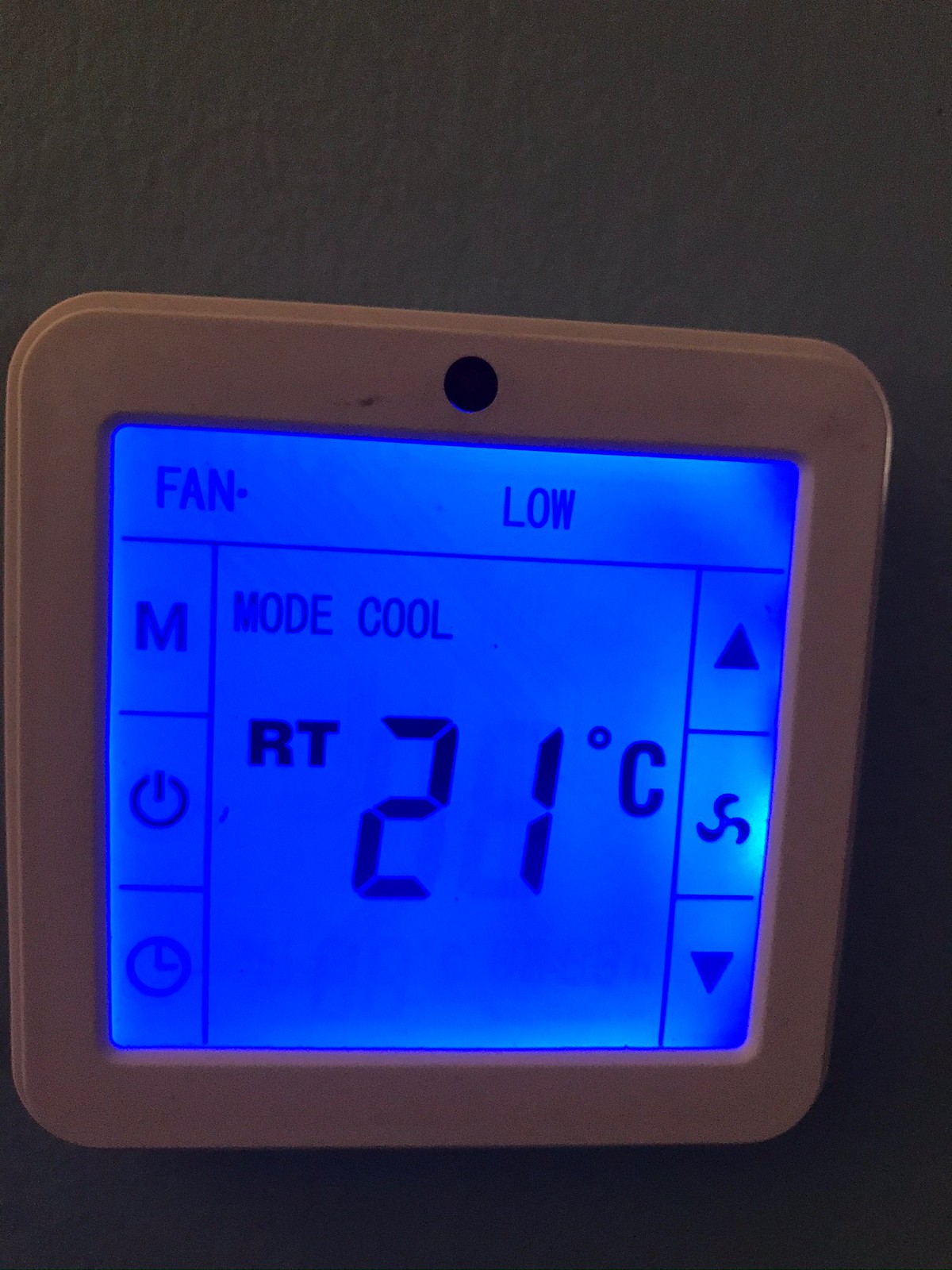The photograph features a contemporary square thermostat prominently mounted on a white wall, occupying most of the frame. The thermostat is mostly white with a central black circle at the top, appearing sleek and modern. The display screen is illuminated in blue, indicating activity. 

In the top left corner of the screen, the word "Fan" is visible, followed by the word "Low" in the top middle. Below "Fan" on the left side is the letter "M," and beneath that is a power icon and a clock icon. The center of the screen displays a box with the text "Mode: Cool," while below that, it reads "RT 21°C," indicating the room temperature setting of 21 degrees Celsius. On the right side of the screen, there is an up arrow, a fan symbol, and a down arrow arranged vertically, likely for adjusting settings.

Notably, there is no visible logo or brand name identifying the manufacturer of the thermostat. The device appears to serve the function of controlling a heating or cooling system.